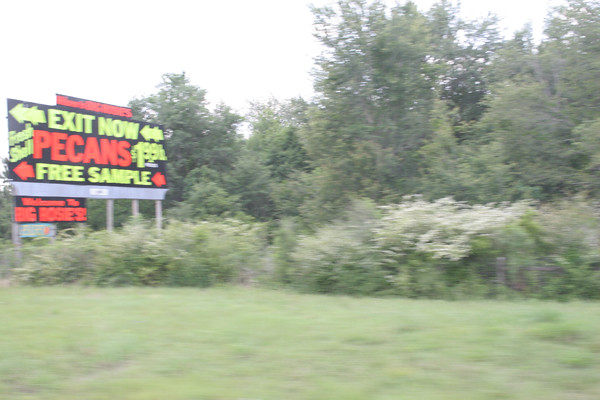A blurred outdoor photograph taken from the passenger seat of a car captures a pastoral scene with a grassy field extending to the middle ground, bordered by a line of dense bushes and towering trees. The sky above is diffuse and gray, casting a muted light over the scenery. On the left edge of the photo, a vividly colored billboard stands out against the natural backdrop. The billboard has a black background with bold yellow and orange lettering that reads, "Exit Now, Pecans, Fresh Shell, $1.99 a Pound, Free Sample." Bright orange and yellow arrows point left, directing attention. Below, a smaller billboard conveys a welcoming message that begins with "Welcome to Big," though the remaining text is obscured due to the photo's blur.